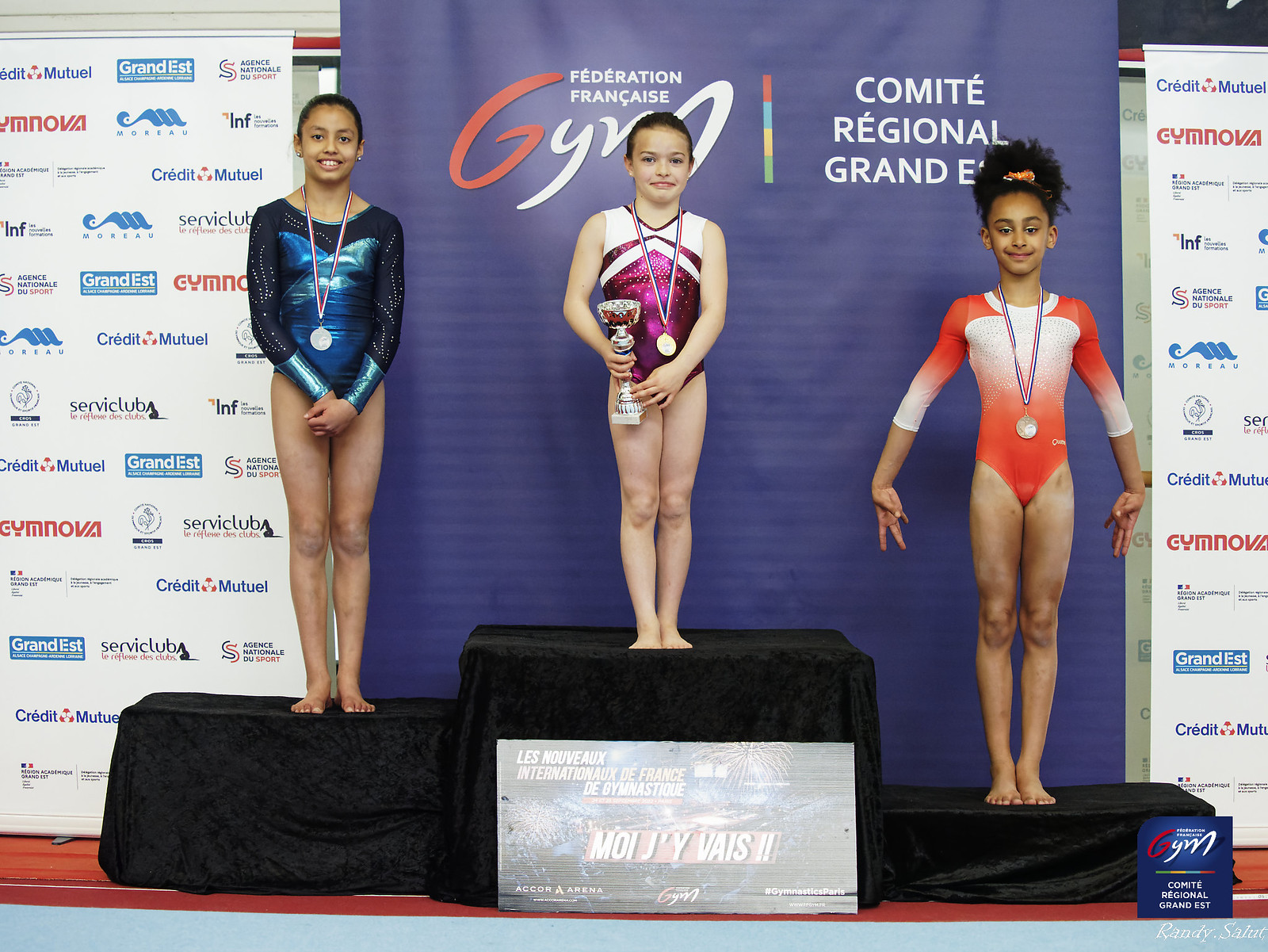The image showcases a vibrant indoor award ceremony for young gymnasts, set against a backdrop of sponsor banners and the Federation Française Gym Committee Regional Grand emblem. Central to the scene are three young girls proudly standing on a tiered black podium. The first-place winner, positioned in the middle and slightly elevated, wears a purple leotard and holds a trophy while also displaying a medal around her neck. To her left, the second-place gymnast is distinguished by her blue and black leotard and similarly adorned with a medal. On the right, the third-place athlete sports an orange and white leotard, also with a medal. The backdrop includes white banners on either side with sponsor names like Credit Mutual, Grand Establishment, and Service Tub, though some are indistinct. The scene captures the celebratory spirit of the event and the youthful pride of the winners.